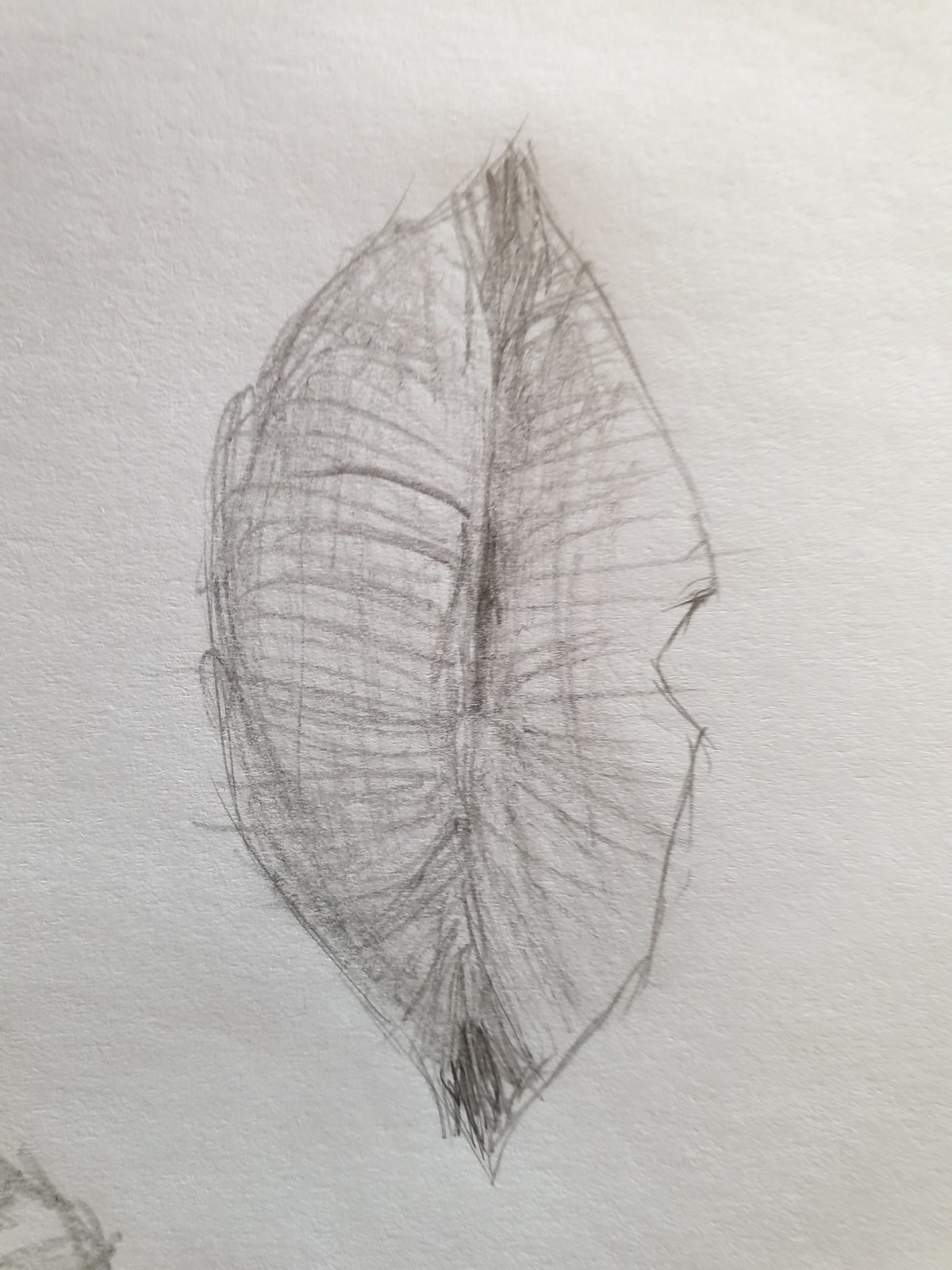This vertical, rectangular sketch appears to depict a pair of sideways lips on a piece of textured cream-colored paper, giving it an artistic and somewhat rustic feel. The lips are oriented with the top lip forming a distinctive V-shape under where a nose would be, extending out widely to poignant corners, then curving into a semicircle underneath for the bottom lip. Heavy pencil lines detail the lips, accentuating the center seam and darkening the corners to enhance realism and depth. The shading is particularly pronounced in the center and at the edges, contributing to a three-dimensional effect. Notably, in the lower left-hand corner of the paper, there seems to be an additional pencil marking, hinting at another drawing or a signature.